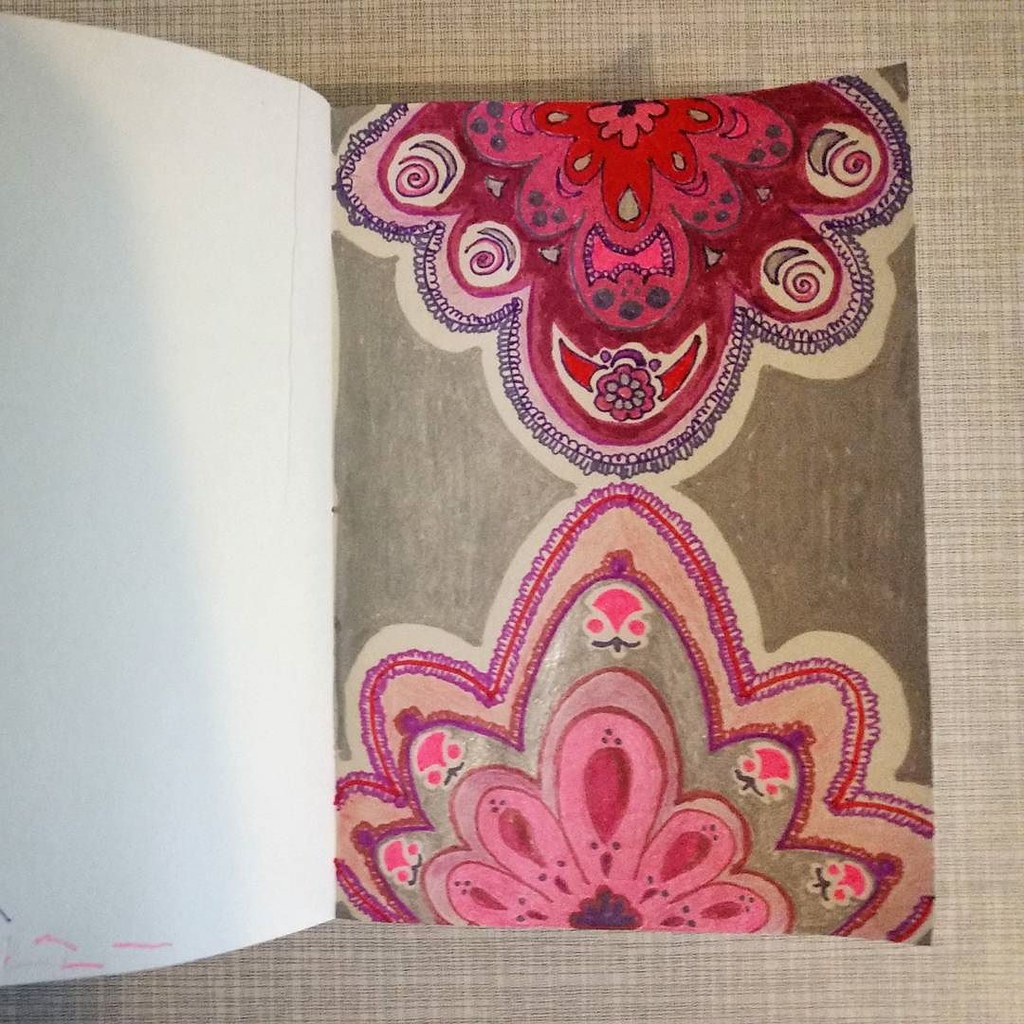This photograph captures the inside of an open journal or sketchbook. The left page is entirely blank, though there's a small blotch of pink ink in the bottom corner, suggesting some color has bled over. The right page features a vibrant, intricate illustration, possibly rendered with markers. The artwork showcases two flowers, mirrors of each other yet distinct, predominantly in shades of pink and purple. The flowers are detailed with various layers, creating a dynamic and colorful composition. The piece seems to be a casual, perhaps amateur, creation rather than a professional one. The journal rests on a beige, checkered linen tablecloth, adding a textured and cozy background. There are no texts or figures in the image, making it challenging to determine the exact notebook size.